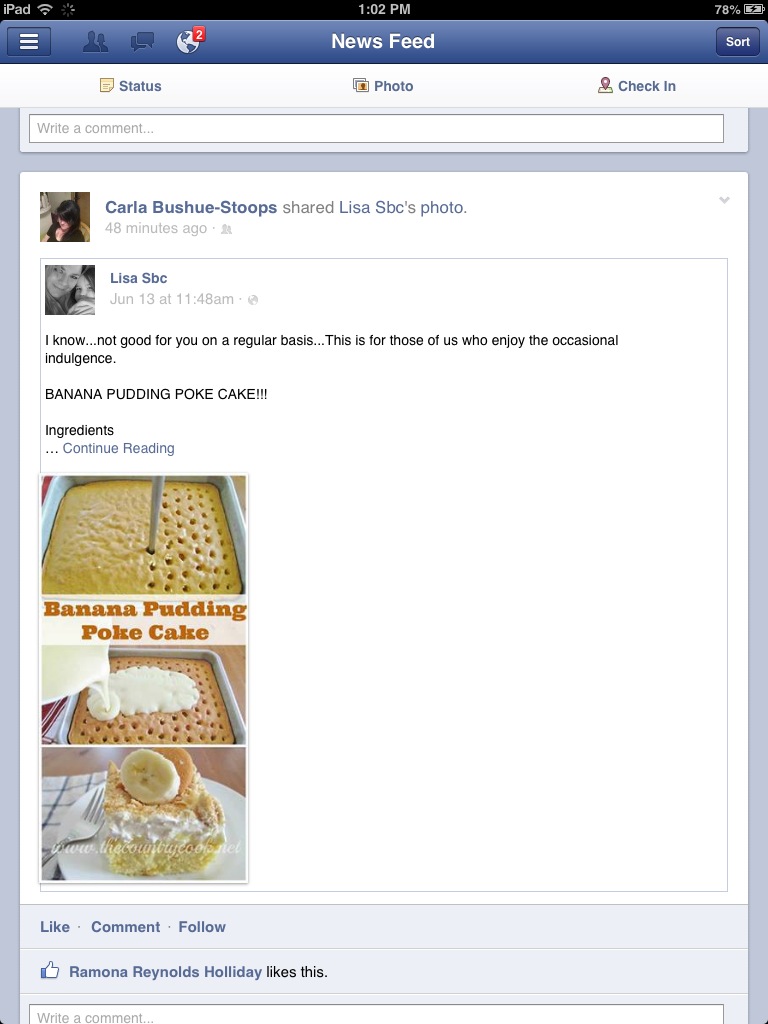This is a tall rectangular screen capture from an iPad, displayed at 1:02 PM with a battery level of 78%. At the top, within a thin black line, it reads "iPad." Below, a thicker blue bar features the text "News Feed" in white. This is followed by navigation options labeled "Status," "Photo," and "Check-In" on a white background.

The main body of the screen shows a Facebook post. In the upper left corner, there is a color profile picture of a woman with long, straight brown hair, identified as Carla Bushu Stoops, next to her name in blue. Below Carla’s name, there is a smaller black and white thumbnail image of a woman hugging a young girl, who is identified as Lisa SBC, also in blue text. The post they shared is dated June 13th at 11:48 AM.

The post's text, in black, reads: "I know… not good for you on a regular basis… This is for those of us who enjoy the occasional indulgence. Banana pudding poke cake." Below this caption, multiple images are displayed: a banana pudding poke cake with yellow filling and poke holes, accompanied by another picture of the cake with frosting on top. The detailed visuals of the cake emphasize the post's indulgent nature.